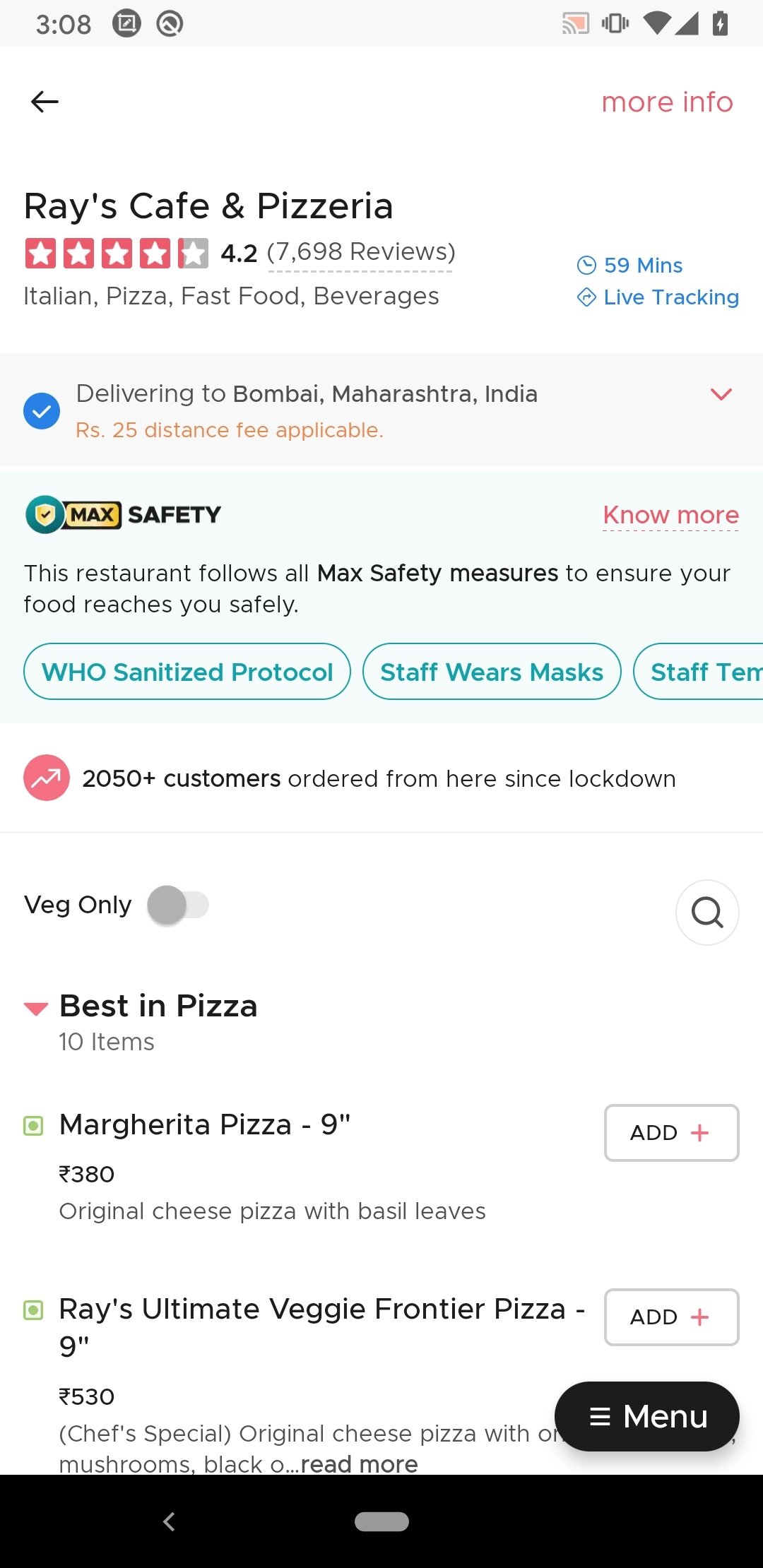**Detailed Caption for the Screenshot:**

The screenshot displays a food delivery app interface at 3:08 PM. The status bar shows two unfamiliar notifications along with other standard icons. The featured restaurant is "Ray's Cafe and Pizzeria," boasting a rating of 4.2 out of 5 stars based on 7,698 reviews. The stars are visually represented with 4.2 out of 5 stars filled in red, while the remaining stars are white. The restaurant offers Italian cuisine, fast food, and beverages. 

Key details include:
- Live Tracking of orders
- 59 minutes estimated delivery time
- Delivery location: Bombay, Maharashtra, India
- A Rs 25 distance fee applicable
- Prominent "Max Safety" measures indicating adherence to WHO-sanitary protocols: all staff wear masks and the restaurant ensures sanitized handling.

Highlighting its popularity, 2,050 customers have ordered from this restaurant since the lockdown began. 

The menu showcases Ray's specialties:
1. Margherita Pizza (9 inches) with an original cheese topping and basil leaves priced at Rs 380.
2. Ray's Ultimate Veggie Frontier Pizza for Rs 530, featuring the chef's special toppings of original cheese, mushrooms, and black olives.

This thorough and informative snapshot concludes with a courteous remark, "Thank you for watching."